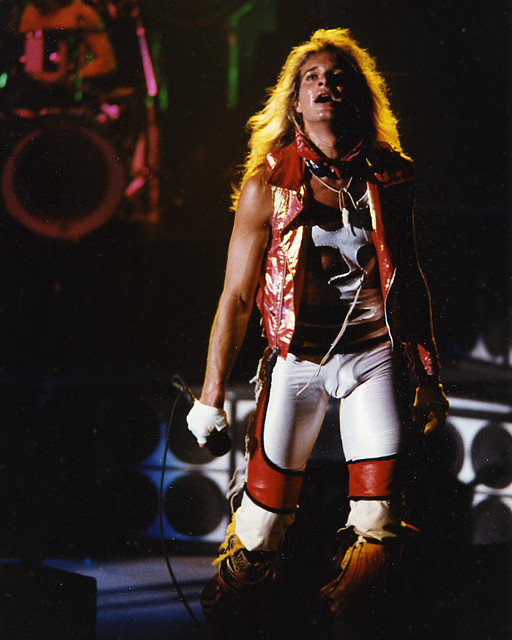This image captures a dynamic scene of a rock star singer on stage, likely David Lee Roth, based on his iconic style. Positioned just right of center in the frame, he is facing forward and looking slightly upward, his long, feathered blonde hair illuminated by stage lights. He is holding a microphone with his right hand, which is gloved in white, adding to his theatrical presence.

The singer is adorned in a striking outfit: a white shirt accented with orange and black, topped by a shiny red and yellow vest. Around his neck is a noticeable red bandana. His white, tight-fitting pants feature bold orange stripes running down the sides, wrapping around his knees, and red bands above the knees, with a distinctive cutout in the crotch area. Completing his look, he sports black boots embellished with yellow tassels.

The stage behind him includes various musical instruments and a drum set, as well as large speakers, hinting at the energetic performance unfolding. The lower part of the image is marked with a patterned white surface featuring black dots, enhancing the visual texture of the scene. Overall, the photograph is a vivid portrayal of a flamboyant rock performance.